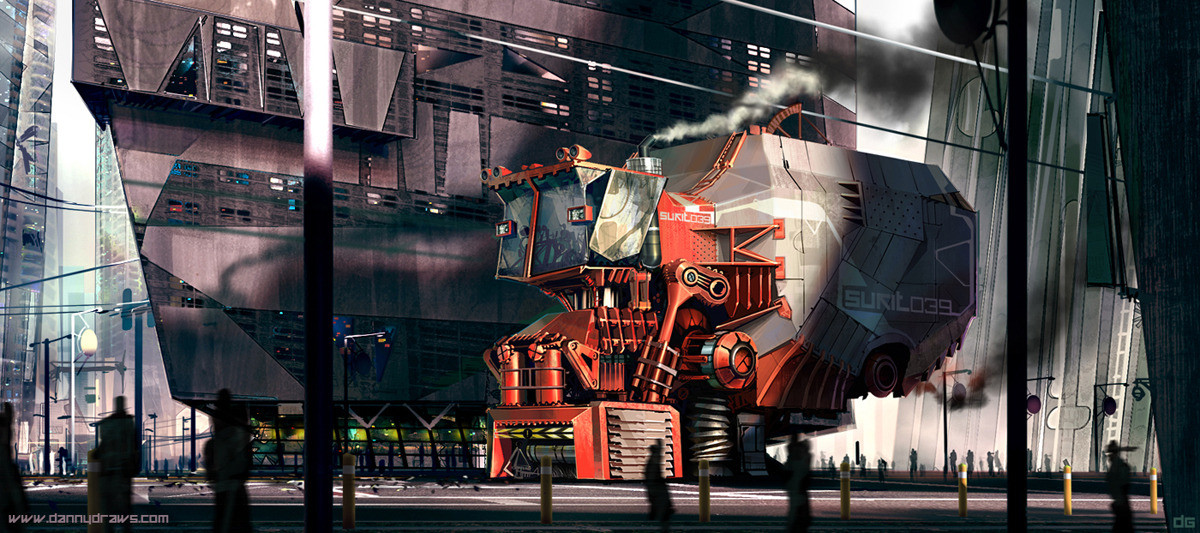The image showcases a detailed, computer-generated, steampunk-style digital painting, prominently featuring a fantastical futuristic garbage truck. This truck is vibrant red, closely resembling a fire engine's hue, and bears an almost anthropomorphic appearance with eye-like features. It is equipped with complex mechanical arms that seem capable of extending and retracting, and there's a ladder along its side. The truck's front end sports a paneled windshield and a smokestack emitting smoke, further enhancing its industrial aesthetic. The scene takes place in an ultra-modern city, characterized by tall, angular buildings, including a remarkably thin structure scarcely a couple of inches thick. The largest building in the backdrop is a grotesque, cut-angled gray edifice with oddly shaped windows, enhancing the futuristic yet eerie ambiance. Scattered throughout the scene are indistinct figures, possibly people, and a smattering of objects that could be dirt or pigeons. The overall composition is vivid and highly detailed, reminiscent of animated movie visuals. At the bottom left of the image lies a watermark that reads www.dannydraws.com.